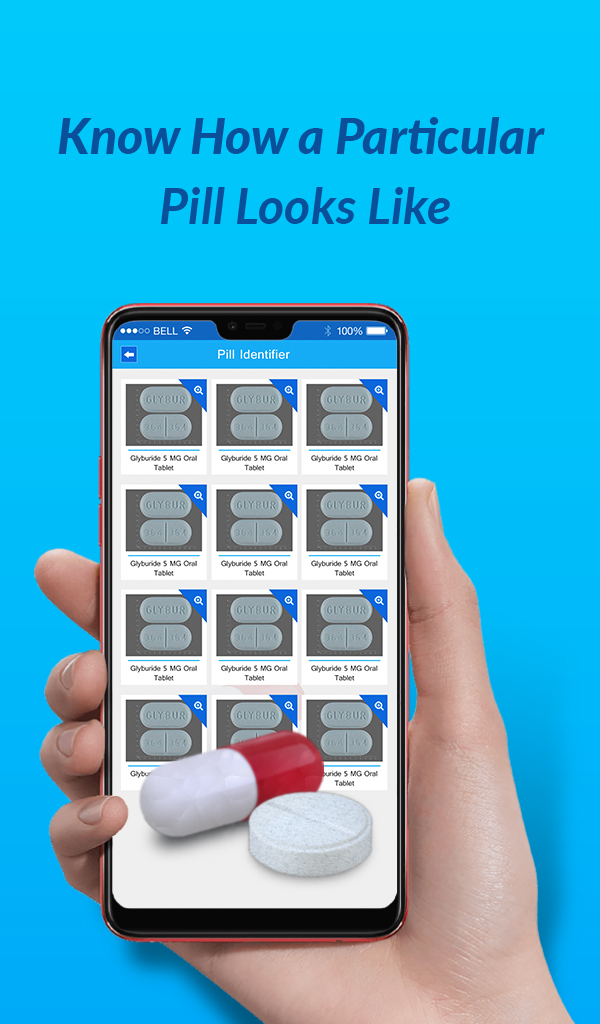A promotional poster showcases the Pill Identifier app against a serene light blue background. In the foreground, the right hand of a woman, perfectly manicured, holds up a smartphone. The phone screen prominently displays the app, which is identified as "Pill Identifier." The app interface currently under development, exhibits repetitive placeholders: identical 5mg oral tablets labeled as Glyburide. Each Glyburide pill is depicted in a grid format comprising four rows and three columns, revealing both the front (with the name) and the back (with a numeral identifier). At the bottom of the phone screen, a larger view highlights an individual pill and another distinct tablet, though its details remain unspecified. The poster effectively illustrates the app's core function, aimed to swiftly and accurately identify unknown pills for users.